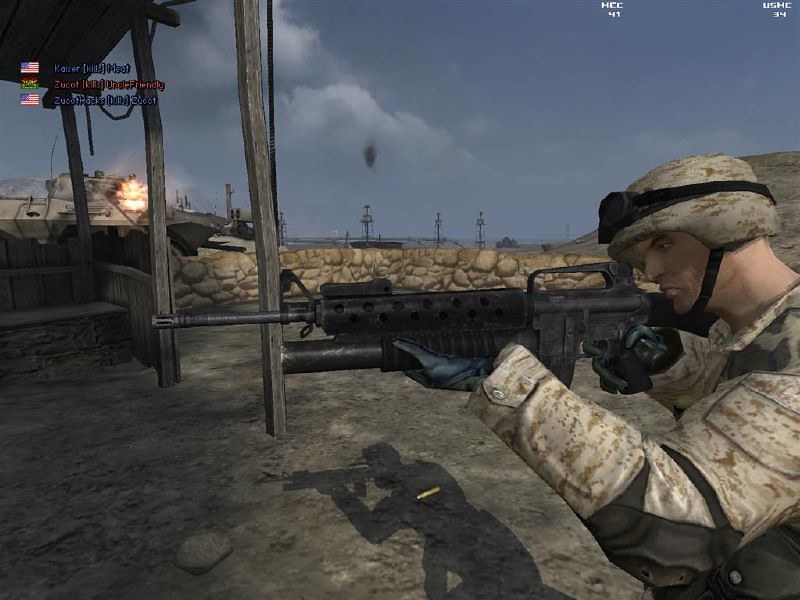The image is a color screenshot from an older-style military-themed computer game. It captures a soldier dressed in camouflaged attire, primarily tan and oily green, crouching behind an olive-tan stone retaining wall. The soldier, a light-skinned man, is equipped with an assortment of gear including a helmet with a black strap under his chin, black gloves, black objects strapped over his elbows, and dark-colored goggles on his helmet. He grasps a black assault rifle with both hands, with one black shell seen flying out of the gun, while another lies on the dirt floor below. 

In the background, a tank is discharging a round, evidenced by the orange muzzle flash. The scene also features a cloudy sky with some visible clouds. The top left corner of the image shows American flags and red and blue fonts, possibly indicating player names or scores such as "MCC 41" or "US HC 34." Notable details also include the soldier's shadow reflected on the ground, adding to the depth of the scenery. Wooden sticks or poles jut out from the stone wall, suggesting a rudimentary structure or roof.